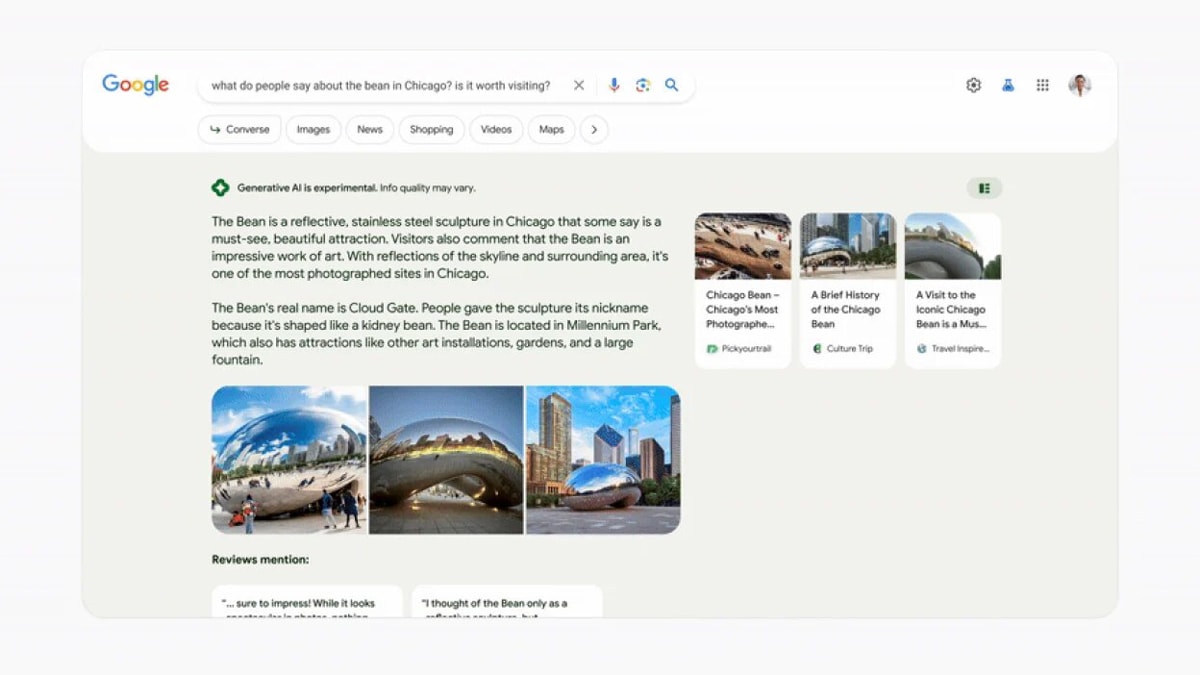This is a screenshot capturing Google search results. The background features a gray tone, and within the main frame is a beige-colored rectangle. At the very top, a thick white bar spans across the screenshot. In the top left corner of this bar, the iconic multicolored Google logo is clearly visible. To the right of the logo, there is a search bar containing text that is too small to decipher. Additional icons are aligned on the far right side of this white bar.

Positioned directly below the search bar is a menu with oval-shaped bubbles, each labeled with different categories such as "All," "Images," "News," "Shopping," "Videos," and "Maps."

Further down, beneath this menu, there is a green diamond icon with a white figure or symbol inside it, accompanied by bold black text to the right of the icon. Following this, two paragraphs of black text are displayed, likely providing context or information about the search query.

At the bottom section, there is a horizontal row featuring three thumbnails of photographs. Each photo provides visual content related to the search. On the right-hand side, at the top, there are three rectangular blocks, each containing a photo at the top with black text below it. The text throughout the screenshot is too small to be read clearly.